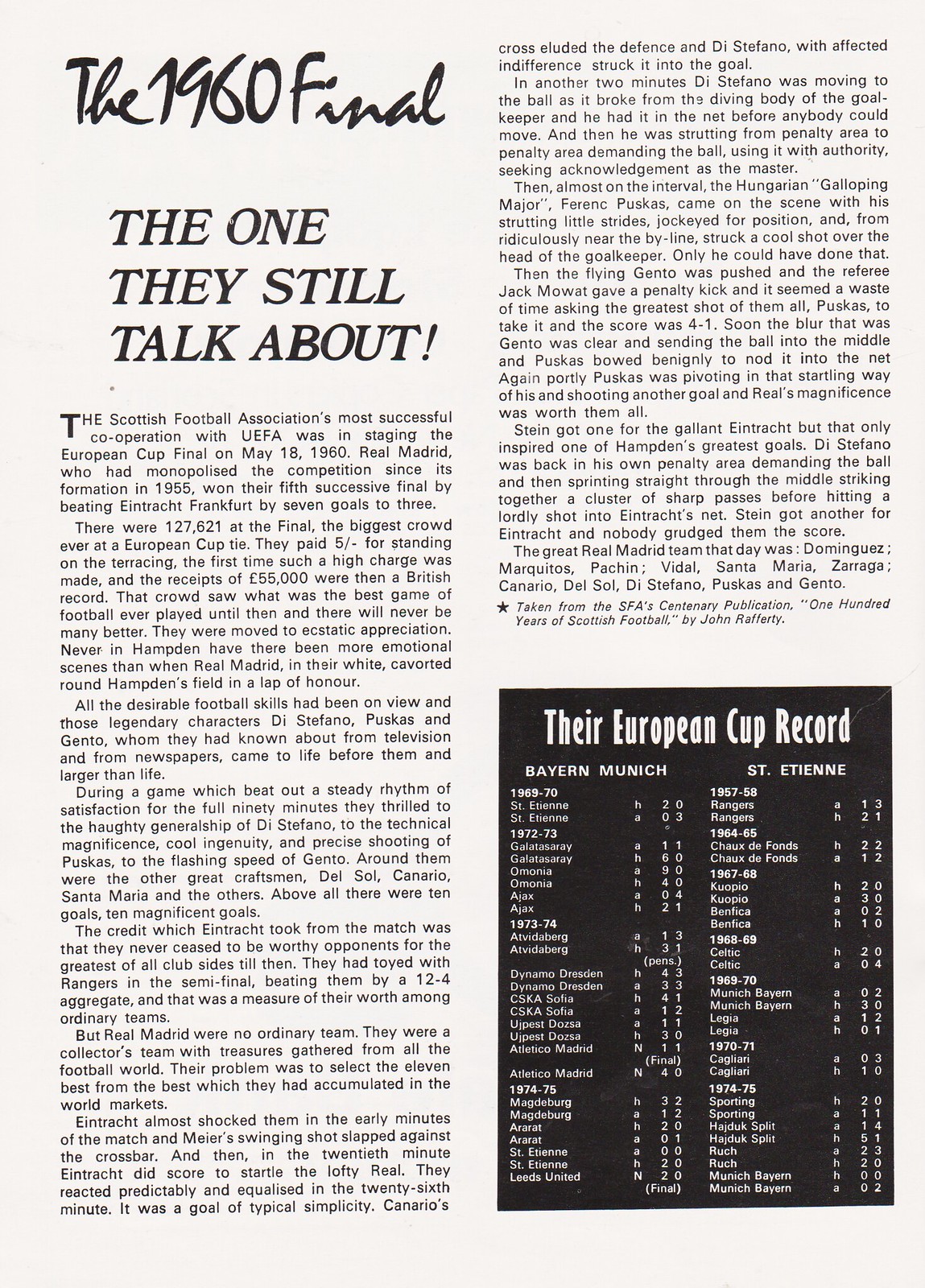The image depicts a magazine page featuring a detailed article about the historic 1960 European Cup final, famously described as "The One They Still Talk About." The page is white, with multiple lines of black text arranged in two columns. The article begins with a heading on the top left corner reading "The 1960 Final." The text highlights the Scottish Football Association's milestone collaboration with UEFA to host the European Cup final on May 18, 1960. This event saw Real Madrid, who had dominated the competition since its inception in 1955, securing their fifth consecutive title by defeating Eintracht Frankfurt with an astonishing score of 7-3. The match set records with an unprecedented attendance of 127,621 spectators, the largest crowd ever for a European Cup tie. This crowd paid a then-record high admission fee, resulting in British record receipts of £55,000. The article emphasizes the unforgettable nature of the match, celebrated by many as the greatest game ever played at that time. Additional details, including a chart on the second column comparing European Cup records of various teams like Bayern Munich and Saint-Etienne, complement the comprehensive recounting of this iconic football event.